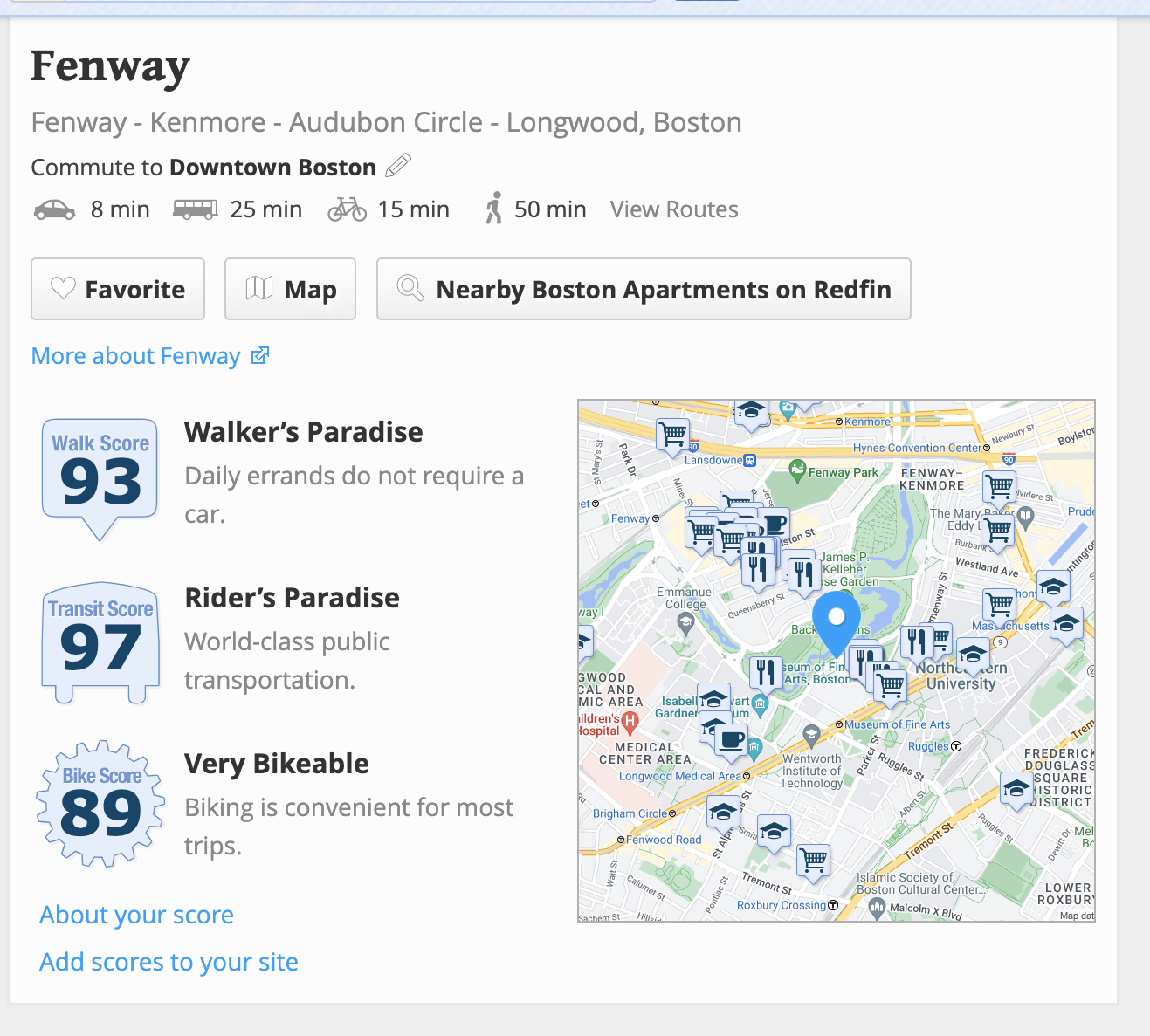**Caption:**
Explore the vibrant Fenway-Kenmore area of Boston, nestled near Audubon Circle and Longwood. This neighborhood offers convenient commuting options to downtown Boston, including an 8-minute ride by pencil, a 25-minute drive by car, a 15-minute bus ride, a 50-minute bike journey, or a scenic walk. 

Discover routes using your favorite maps, and explore nearby apartments listed on Redfin. Fenway boasts a stellar Walk Score of 93, indicating that daily errands do not require a car in this walker's paradise. The Transit Score of 97 reflects world-class public transportation, making it a rider's paradise. With a Bike Score of 89, biking is a convenient option for most trips in this very bikeable area. 

The map features a blue dot at the center, surrounded by icons representing shopping carts, schools, coffee cups, and dining utensils, highlighting the variety of amenities available. This neighborhood truly stands out as an ideal place to live for those seeking a blend of convenience and community.